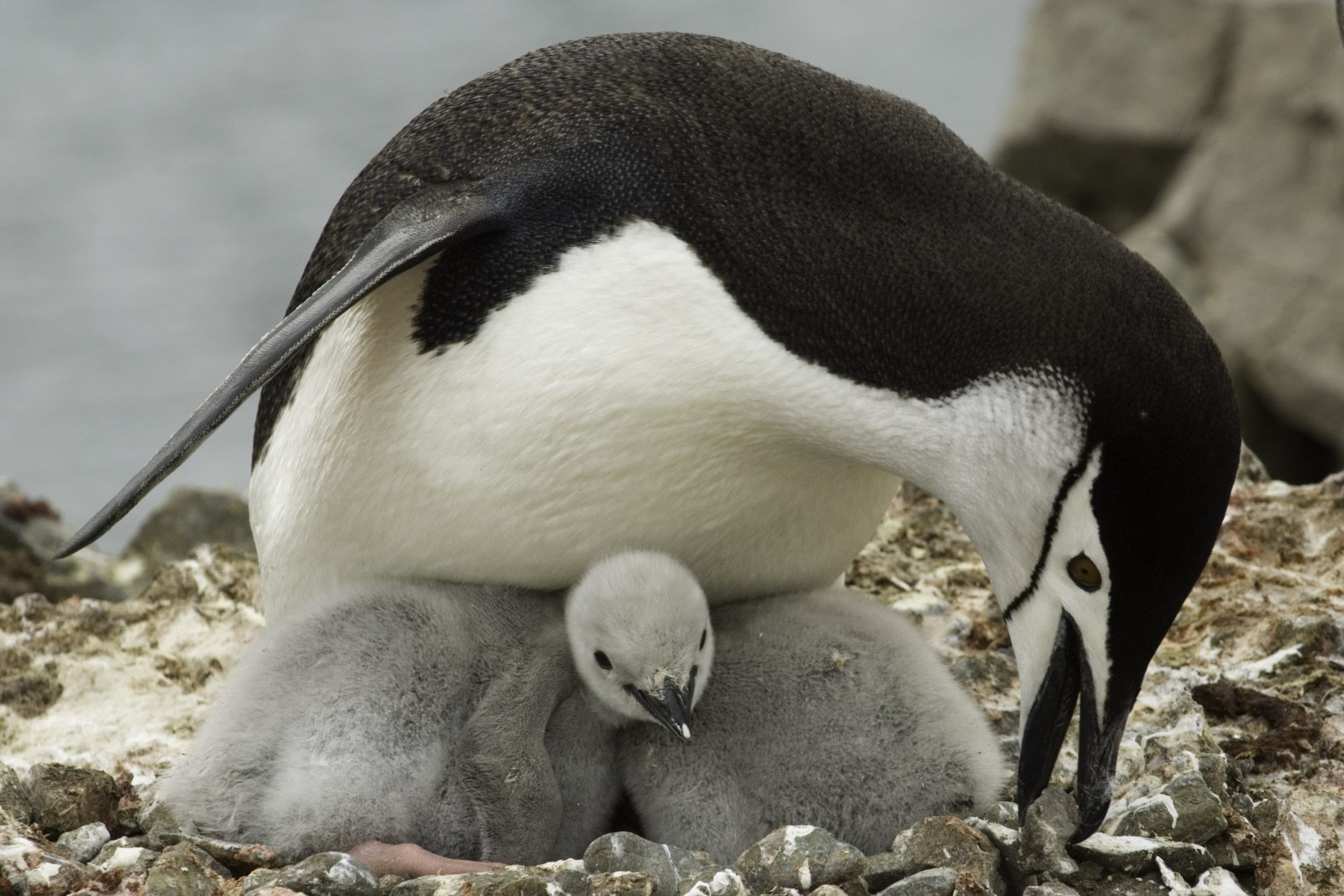In a gray, outdoor setting filled with rocks, sand, and pebbles, a mother penguin with a black back and white chest is hunched over her nest, providing warmth and protection to her young. She is seen picking up a rock with her beak, possibly to fortify her nest. Tucked securely beneath her, one can see the fluffy gray plumage of her babies, yet to develop the distinct black and white tuxedo pattern of their parent. One baby penguin, with its soft white head and black beak, peeks out from between her feet, while the presence of more might be hidden under her protective posture. The background hints at a nearby water source, contributing to the scene's muted, gray atmosphere.